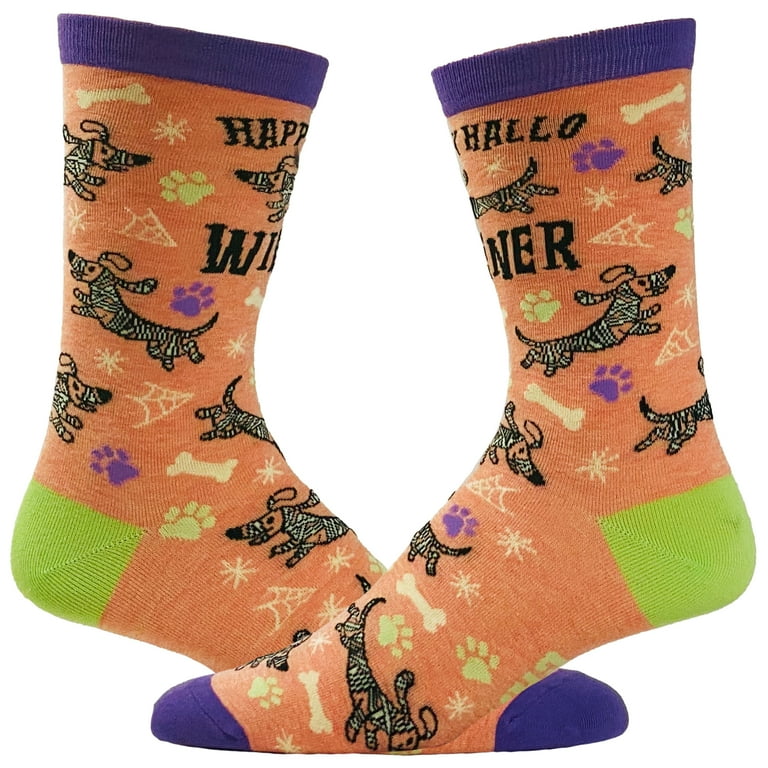This photo features a vibrant pair of shin-length Halloween-themed socks. The main body of the socks is bright orange with intricate designs and text. The heels are light green, and the toes are a dark purple, matched by a purple lining at the top of each sock. One sock's toes point left, and the other points right, both overlapping slightly where the foot would be.

Prominent on the socks is an embroidered image of a playful wiener dog wrapped in what appears to be black and white mummy wraps, complete with a loosely draped leash around its head. The text "Happy Halloweener" is split across the socks, reinforcing the Halloween motif with a playful twist on words. Additionally, the socks are adorned with colorful Halloween-themed patterns, including green and purple dog paw prints, yellow bones, and white spiderwebs. The overall effect is fun and festive, making these socks a whimsical choice for the Halloween season. The background of the image is solid white, highlighting the vivid colors of the socks.